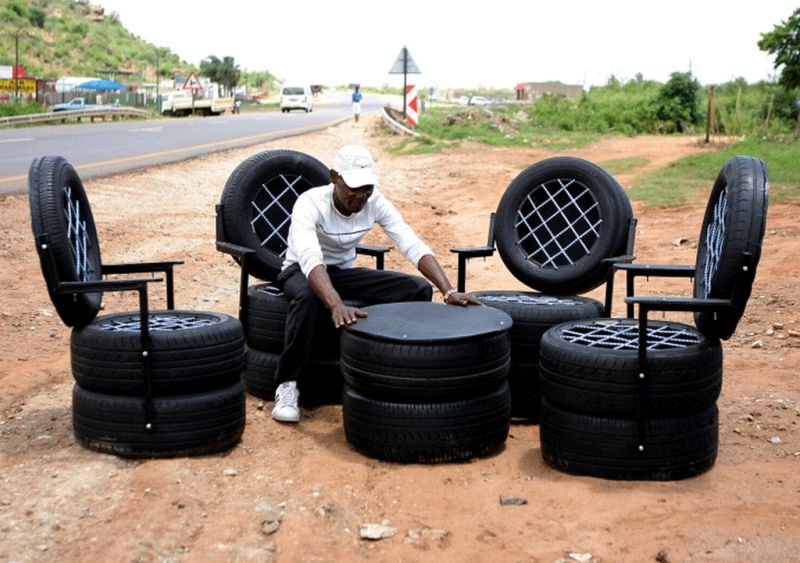In the color photograph, we see a creative and resourceful scene centered around a man sitting on a makeshift chair constructed entirely out of car tires. The backdrop is a wide, dirt-covered spot adjacent to a road that features both moving and parked cars, with a silver metal guardrail marking the edge. The man, identified by his dark brown skin, wears a white ball cap, a white long-sleeved shirt rolled up to his elbows, black pants, and white sneakers. Notably ingenious, he has fashioned four chairs and a coffee table from black rubber tires, each stack meticulously assembled. Two large tires serve as the base of each chair, with an armrest bolted in place, and a smaller tire, incorporating a grill on the back, forms the backrest. The table in front of him is similarly made from stacked tires. The surroundings feature a combination of red, sandy brown dirt and rocks, with greenery such as grass and trees interspersed. A hill covered in green grass rises to the left, while the right side reveals another path. The atmosphere is marked by a cloudy sky, adding depth to the day, and additional details include people walking along the road. This inventive makeshift setup exemplifies utilitarian creativity amidst a backdrop of a rustic, natural environment.